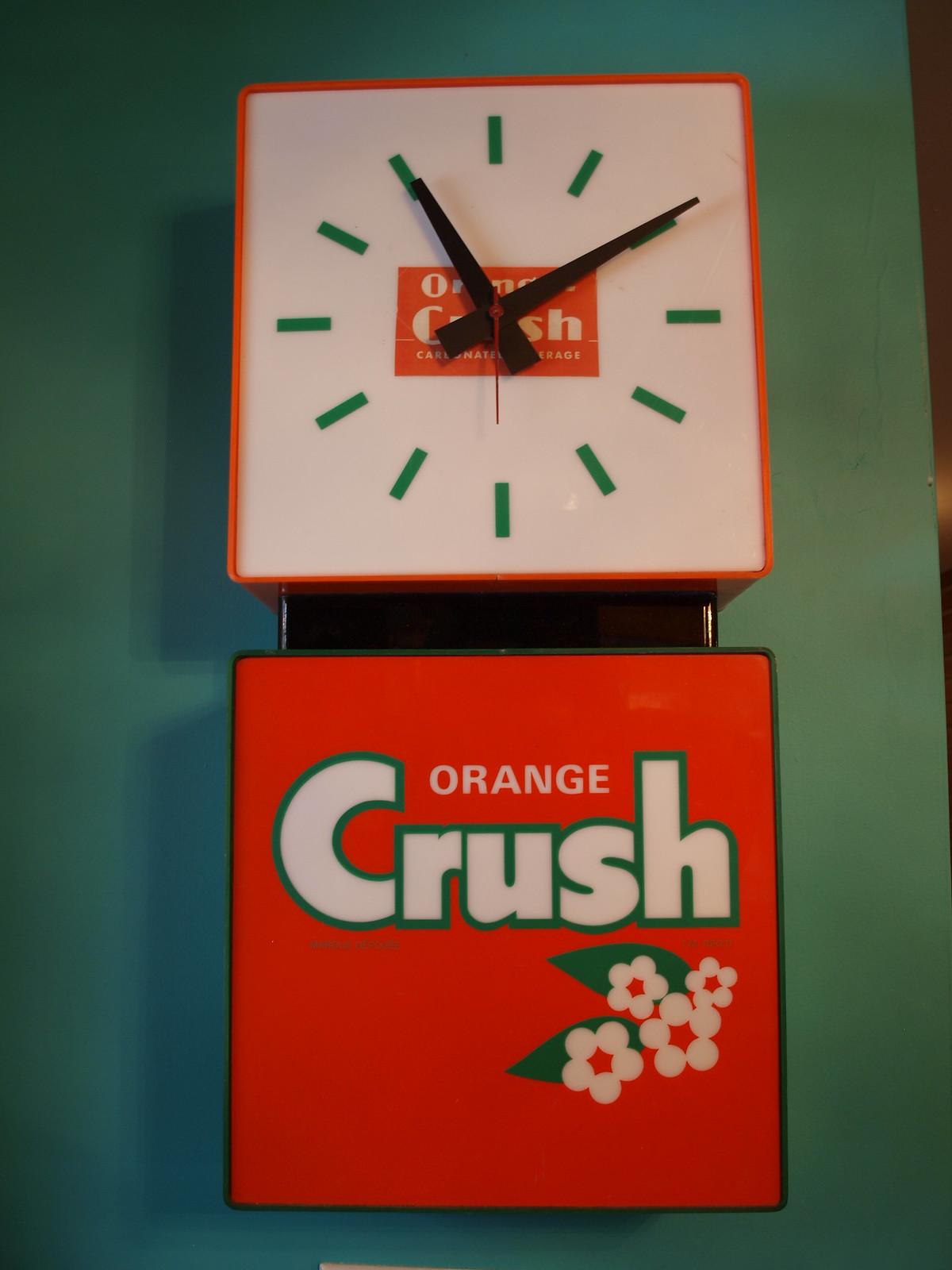This photograph captures a vintage clock mounted on a wall, possibly within a restaurant setting. The wall is painted a dark green hue, which closely matches the green outline of the "Orange Crush" soda logo adorning the clock. The clock itself is divided into two squares: the upper square features the clock face, while the lower square displays the vibrant "Orange Crush" advertisement.

The upper square's clock face is predominantly white, with green hour indicators. At its center, just beneath where the hands are attached, is an orange sign that reads "Orange Crush" in bold, orange letters. The clock's hands are black, except for the second hand, which is strikingly red.

The lower square showcases the "Orange Crush" sign, set against an orange background. This section is accentuated with green leaves and delicate white flowers, adding a touch of natural charm. The word "Crush" is prominently displayed in white, bordered by a green outline. The entire clock is elegantly framed with an orange border around the upper square, harmoniously integrating the overall design.